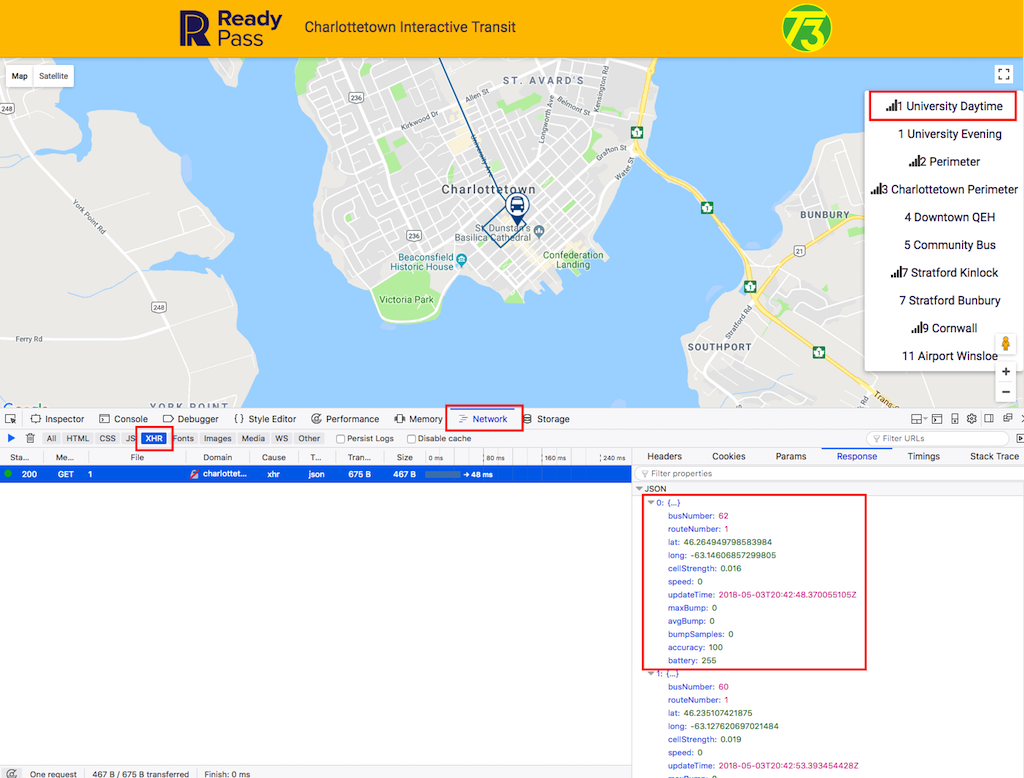The image is a screenshot showcasing the "Ready Pass Charlottetown Interactive Transit" website, revealing both the user interface and underlying code. The upper half depicts a detailed satellite map of Charlottetown, featuring a transit icon and a comprehensive menu on the right listing various transport routes such as University Daytime, University Evening Perimeter, Charlottetown Perimeter, Downtown QEH, Community Bus, Stratford Kinloch, Stratford Bunbury, Cornwall, and Airport Winslow. 

The lower half is a glimpse into the developer's workspace, split into two sections. The left section displays the current file name, while the right section showcases lines of code. Certain parts of the code are emphasized with a red outline, likely indicating areas of interest or concern. Additionally, multiple tabs are visible at the top, with "Network" and "XHR" highlighted in red, suggesting active debugging or network inspection. The top portion of the coding area is also contained within a red box, further marking significant segments. This dual-view illustration underscores both the functional and developmental aspects of the transit website.